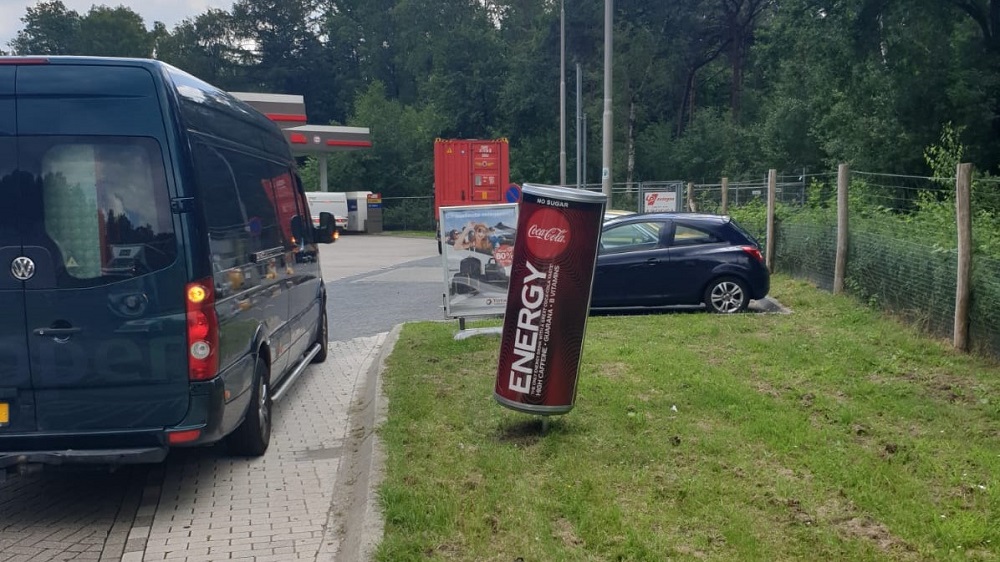The image captures the front entrance of a typical gas station or rest stop. Dominating the center is an advertisement featuring a large, red can designed to look like a Coca-Cola energy drink, complete with the familiar logo and the words "Energy" and "No Sugar" displayed prominently. To the left of this advertisement, a dark blue Volkswagen van is seen entering the parking area, accompanied by a black hatchback vehicle and a red truck in the background. The right-hand side of the image shows a green, grassy area bordered by a concrete edge, with an adjacent wire fence supported by wooden posts, marking the boundary of a wooded area. Behind the main Coca-Cola ad, another sign depicts a scenic mountain view in a vertical format.